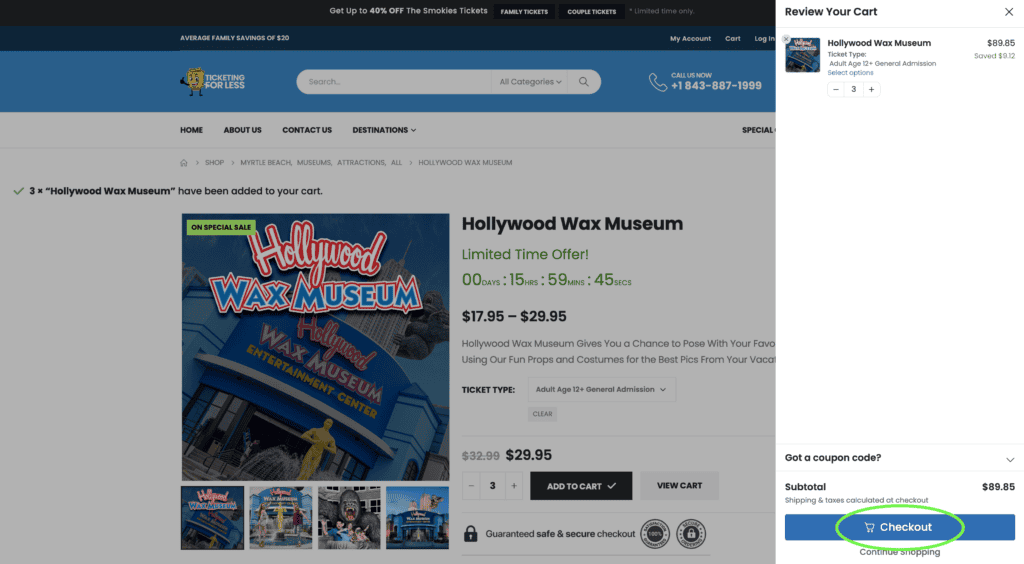**Caption:**

An online checkout screen for the Hollywood Wax Museum showcases a vibrant and detailed shopping experience. The page prominently features a package for the Hollywood Wax Museum, highlighted by bold white text with red accents and a distinctive blue wax font with a red and white outline. The museum’s Entertainment Center is spotlighted alongside an enticing sale banner with a countdown timer reading 0 days, 15 hours, 59 minutes, and 45 seconds, emphasizing the urgency of a limited-time offer.

Displayed prices range from $17.95 to $29.95, with a descriptive note inviting visitors to pose with their favorite figures using fun props and costumes—ideal for capturing memorable vacation photos. The ticket type listed is for general adult admission at $29.95 with options for different ages.

The cart summary, located at the top of the page, details the purchase of three general admission tickets for those aged 12 and over, totaling $89.95 with a noted saving of $9.12. A customer service contact number, 843-887-1999, is positioned at the top right, and a prompt to review the cart sits beside it. Below, there is a space to enter a coupon code, indicated by a downward-pointing triangle. The subtotal is displayed as $89.85, with a reminder that shipping and taxes will be calculated at checkout. Finally, a green-encircled "Checkout" button stands ready for the next step in the purchase process.